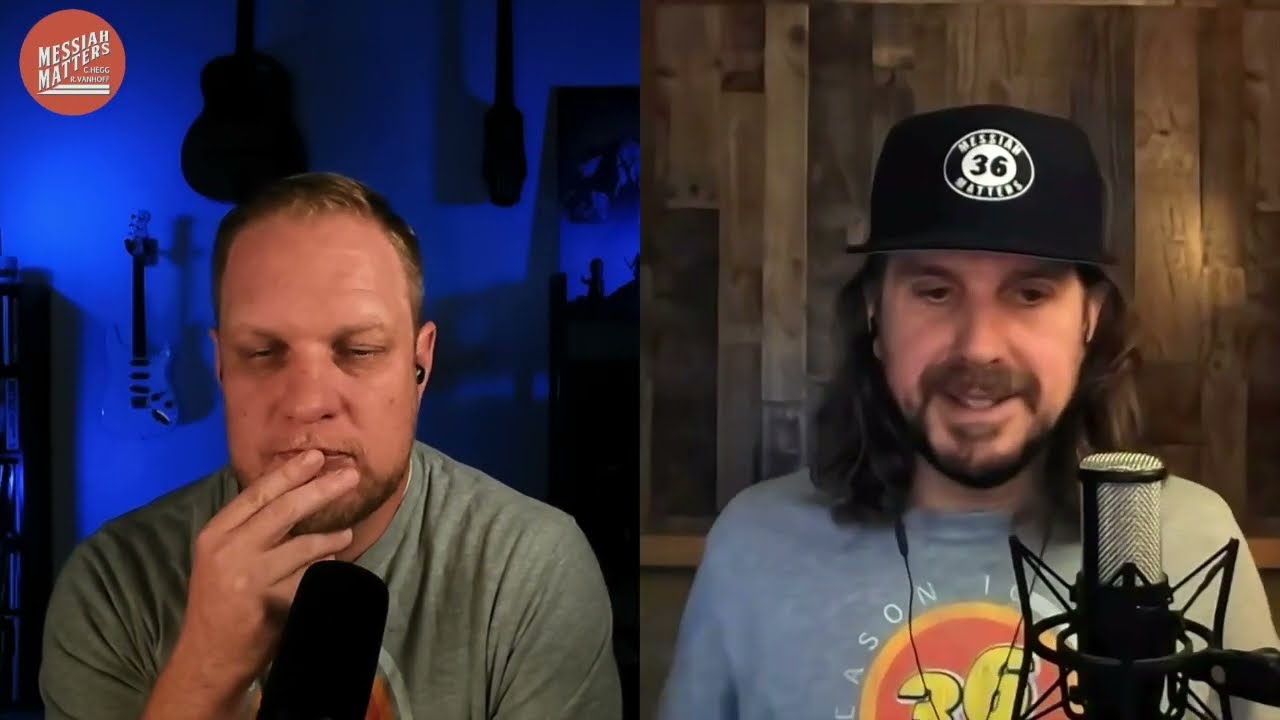This image is a horizontal rectangular photo of two men engaged in a podcast, each speaking into a microphone. The man on the left has very short blondish-brown hair and is wearing a greenish T-shirt. He has an earbud in his left ear, and his hand covers his mouth while a black microphone stands in front of him. The background behind him features blue lighting with a dark tone, and in the upper left-hand corner, the text "Messiah Matters" appears in white letters within a circle. The man on the right, situated in front of a wood panel wall, dons a black flat-brim cap with the number 36 in yellow. He has shoulder-length shaggy brown hair, a brown mustache, and a beard. He is dressed in a gray T-shirt with a graphic print featuring the number 36 on it. His silver microphone stands prominently before him. Behind the two men, several guitars hang on the wall, adding to the ambiance of their podcast setting.